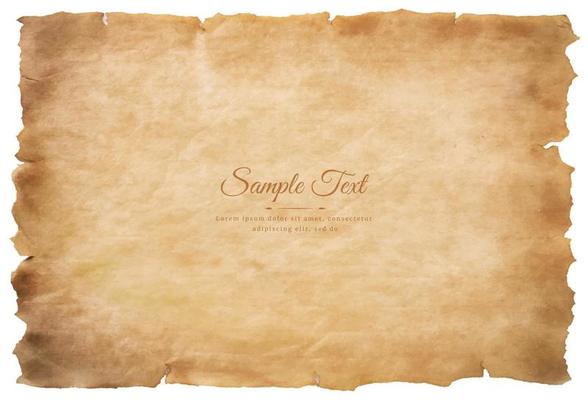The image depicts a rectangular piece of parchment with a significantly aged appearance. The parchment has dark brown, irregular edges as if it has been lightly burned, furthering the worn and ancient impression. The center of the parchment transitions from a darker brown at the borders to a lighter brown, more standard parchment color towards the middle. The phrase "sample text" is prominently displayed in the middle using a script-like font and is underlined. Below "sample text," there is additional, much smaller text that is hard to decipher due to its size and blurriness. The overall texture of the parchment appears cracked and weathered, resembling old, historical documents or ancient scripts. This aged document appears to serve as a template or backdrop, possibly for an illustrative or informative purpose.